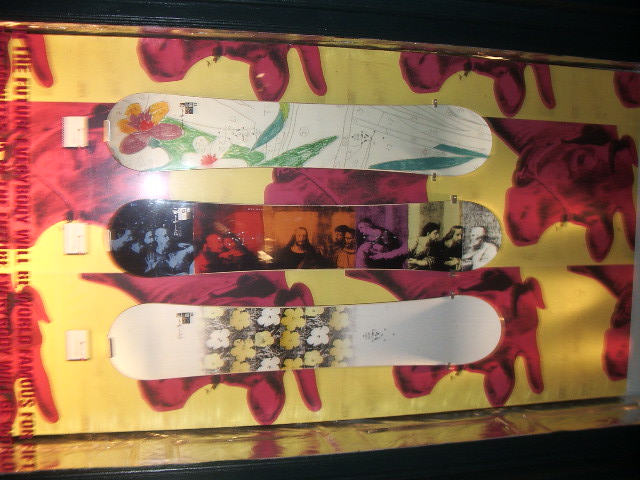This landscape color photograph captures a mounted display of three skateboards, though it lacks sharpness and clarity. The background, poorly focused, features a yellow and red design with obscure shapes, potentially resembling repeated cow heads, though their true nature is indistinct due to the low image quality. The display appears in some form of a cropped, indoor setting, possibly on a wall or within a frame, with vertical text along the left side that remains unreadable.

Positioned horizontally, the skateboards are notable for their artistry. The top skateboard exhibits a hand-drawn, colored pencil design of flowers with green foliage on a white background, showing apparent sketch lines that give it an unfinished look. The middle skateboard is an eye-catching piece, displaying a religious image believed to be Jesus at the Last Supper, overlaid with a spectrum of colors including blue, red, orange, purple, green, and gray. The bottom skateboard, set against a black background, features a central band of detailed white and yellow flowers interspersed with black foliage that contrasts sharply with the vibrant floral pattern.

Despite the blurred, low-quality nature of the photo, the colorful, detailed designs on the skateboards and the visually engaging background make the image rich in context and aesthetic intrigue.